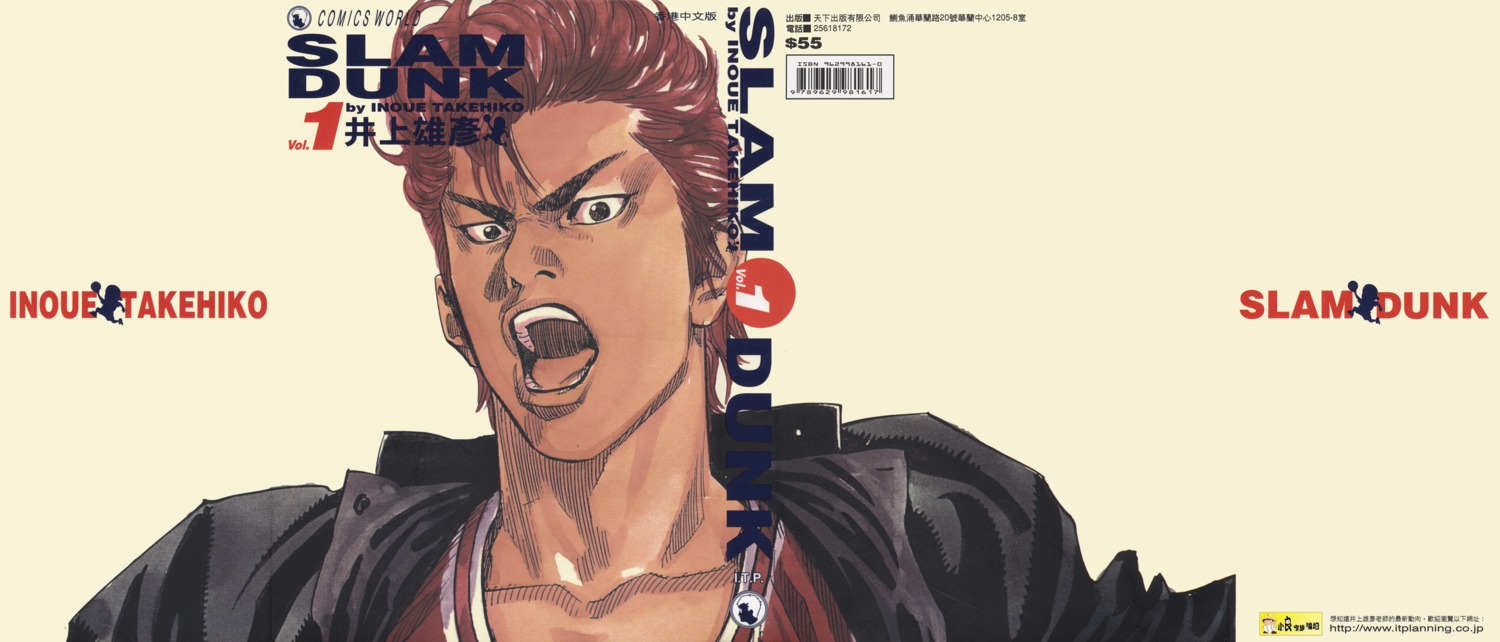This image features a striking cartoon rendition of an angry man, positioned slightly to the left of the center against an eggshell-colored background. The man has olive-colored skin, dark, triangular eyebrows, and a reddish-brown pompadour hairstyle. His mouth is wide open, revealing his white teeth, as if he is shouting. He is dressed in a black leather jacket over a red shirt with white trim, resembling a Chicago Bulls basketball jersey. The text surrounding the figure includes the red-lettered "Slam Dunk" on the right and additional red text that reads "Inui Takahiko" on the middle left. Black letters at the top left spell "SLAM" with "DUNK" below it, alongside Japanese characters. Additionally, there is a red circle with a white "1" next to the man's head, emphasizing the 'Volume 1' label. This combination of vibrant colors, dynamic posture, and stylized text, including "Slam Dunk 1" in black around the head, aligns with a comic book or anime style, possibly indicating a Japanese origin.